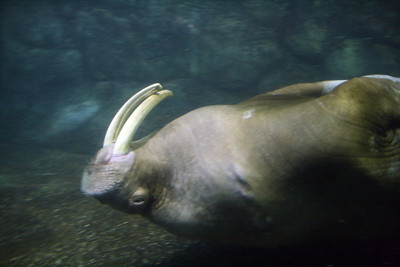This close-up underwater image captures a walrus in a tranquil moment, sleeping upside down. At the top of the image, the dark blue water signifies the aquatic setting, while the bottom showcases the surface, blending from a black hue in the lower right to a lighter brown in the lower left. The walrus's body, with its upper part appearing whitish and its lower part exhibiting a brownish tint with white features, occupies a significant part of the frame, stretching from the right-hand side of the image. The walrus's distinct long white tusks are pointing upward, accompanying its visible nose, eyes, and prominent whiskers. The backdrop suggests the presence of a tank environment, possibly in an aquarium, with hints of rocks behind the creature. The reflection of the water adds a serene element to this captivating marine scene.